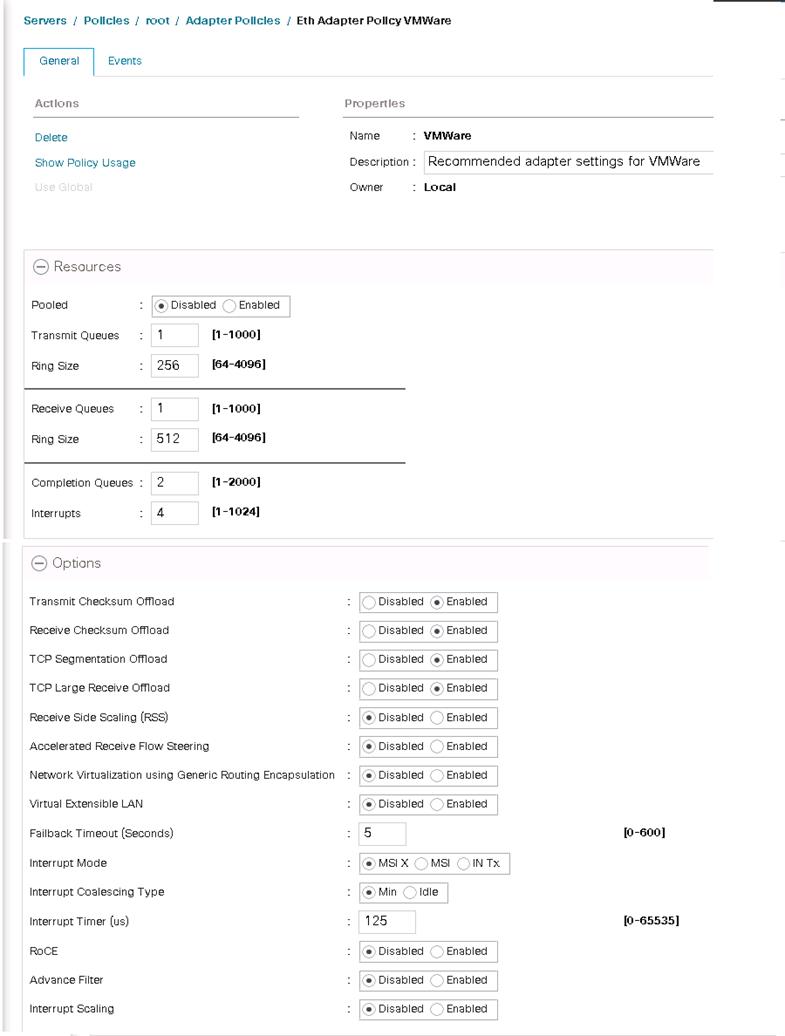The image showcases a VMware settings screen with the user path displayed at the top, indicating navigation through "Servers > Policies > Root > Adapter Policies > Adapter Policy VMware." The screen is focused on the "General" tab, while another tab labeled "Events" is present but not selected.

Under the "Actions" section on the "General" tab, the available options include "Delete," "Show Policy," and "Usage." The "Property" section lists the following details:
- Name: VMware
- Description: [Not specified]
- Owner: Local

In the "Resources" section, several configurations are displayed:
- Status: Pooled (option to select either Disabled or Enabled)
- Transmit Queues: 1
- Ring Size (Transmit Queues): 256
- Receive Queue: 1
- Ring Size (Receive Queue): 512
- Completion Queue: 2
- Interrupt: 4

Under the "Options" heading, the parameters and their current settings are listed as follows:
- Transmit Checksum Offload: Enabled
- Receive Checksum Offload: Enabled
- TCP Segmentation Offload: Enabled
- TCP Large Receive Offload: Enabled
- Receive Side Scaling: Disabled
- Accelerated Receive Flow Steering: Disabled
- Network Virtualization using Generic Routing Encapsulation: Disabled
- Virtual Extensible LAN: Disabled
- Fallback Timeout: 5
- Interrupt Mode: MSIX
- Interrupt Coalescing Type: Min
- Interrupt Timer: 125
- ROCE: Disabled
- Advanced Filter: Disabled
- Interrupt Scaling: Disabled